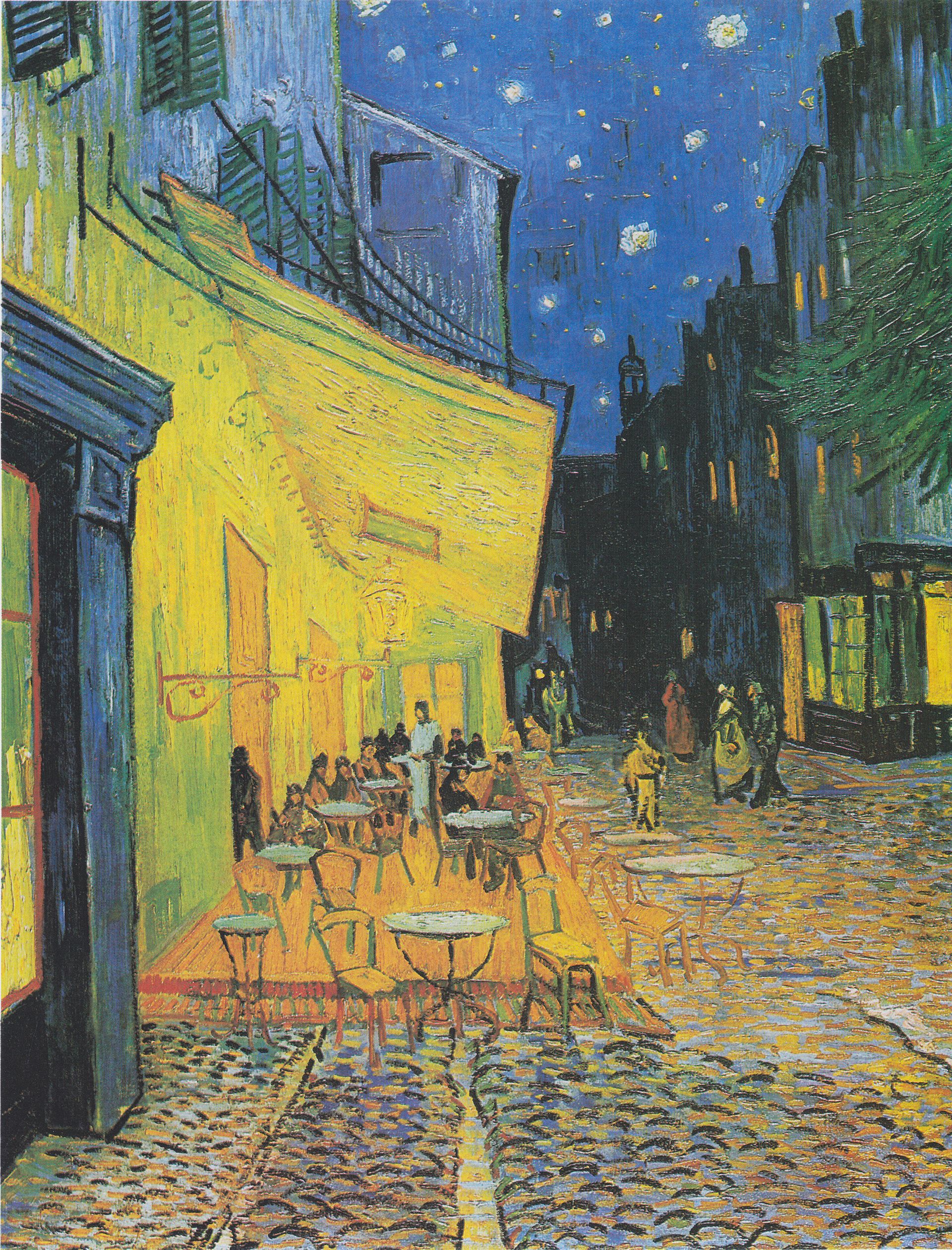This vertically aligned rectangular painting, identified as Vincent van Gogh's "Cafe Terrace at Night," captures a vibrant evening scene in Arles, France. The sky is a deep, starry blue punctuated with white and yellow stars, creating a characteristic Van Gogh-esque swirling effect. The painting showcases a bustling city street at night, featuring a quaint outdoor café with round tables and chairs located in the middle-left portion of the scene. Patrons can be seen sitting at these tables, likely attended by a server, all under a prominent yellow awning. This awning extends from a two-toned building — yellow on top and green below. Adjacent buildings line the street, depicted in darker shades of black and dark blue, contributing to the nighttime ambiance. Tree branches hang into the frame from the upper right, adding a touch of nature to the urban landscape. The cobbled rock walkway in the foreground, with people strolling across it, further enriches the lively atmosphere of this iconic Van Gogh masterpiece.